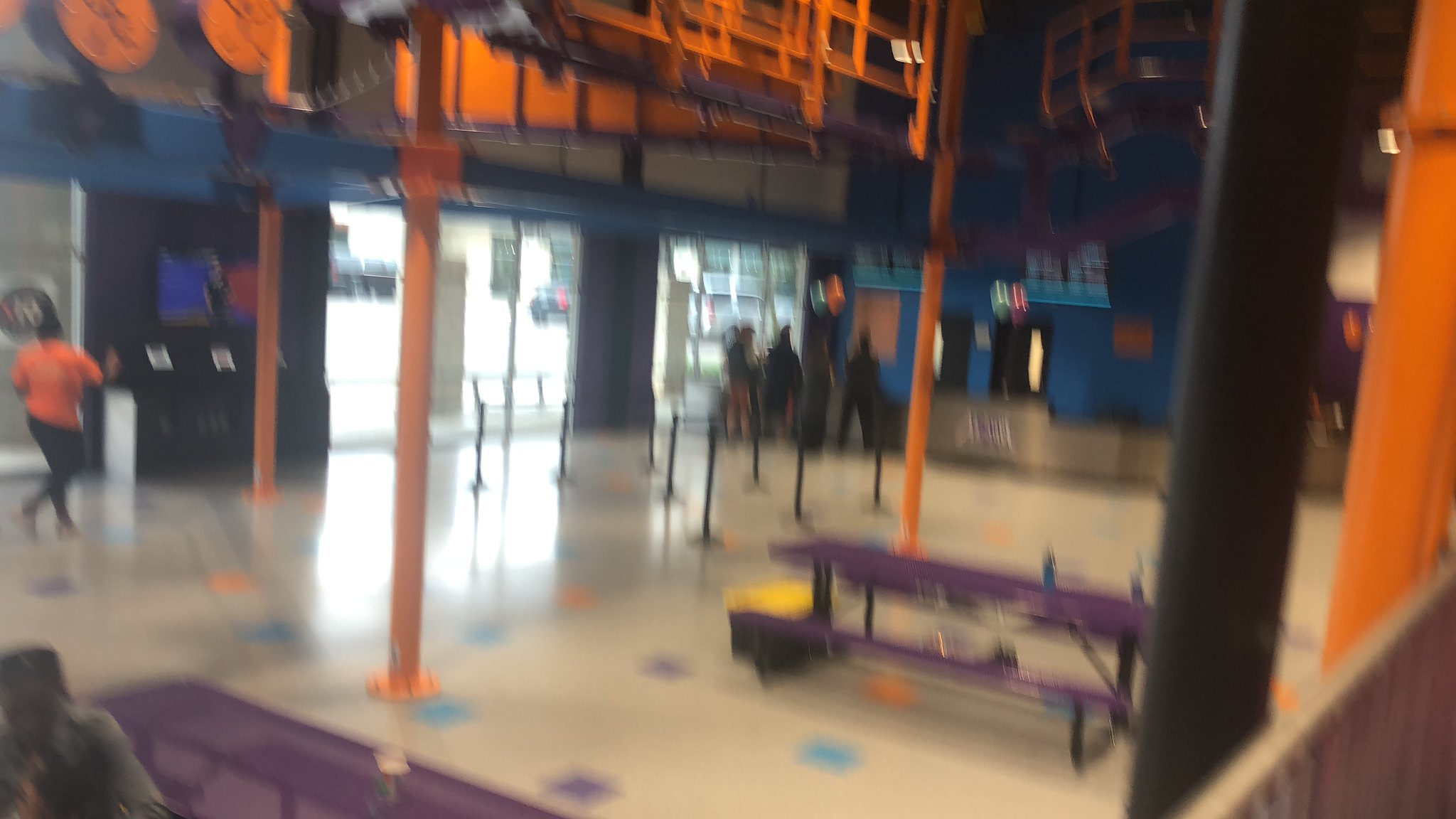The image depicts a vibrant children's activity center, possibly a bounce house or trampoline park. The scene is filled with a lively color palette featuring oranges, purples, and bright blues. A queuing area is visible, suggesting a structured entry process for guests. The facility appears to be relatively empty, likely indicating it is during school hours. Orange poles are strategically placed throughout the venue, adding to the playful environment. Notable elements include a purple picnic table with what seems to be a blue Gatorade bottle on top. Employees dressed in orange shirts and black pants are seen walking around, maintaining the space. At the front, a large blue wall marks the counter where visitors likely purchase their tickets for entry.